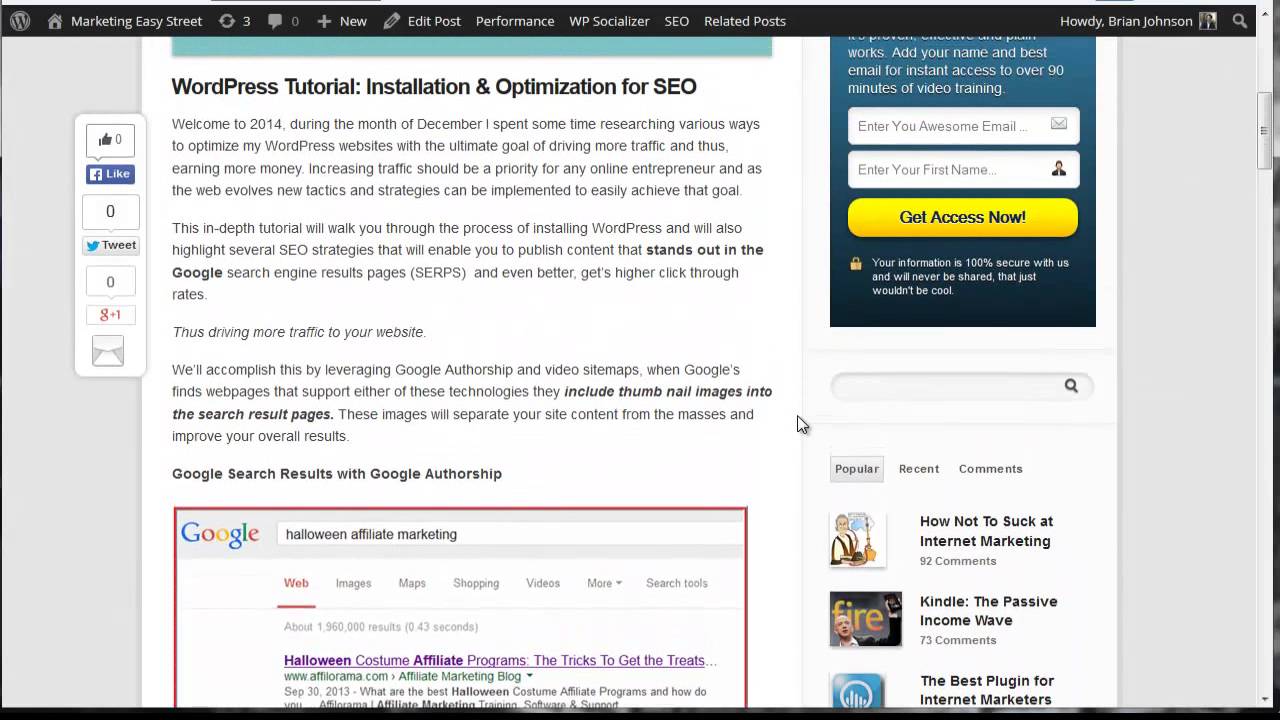### Detailed Caption for the Image:

This image is a screenshot of a computer screen, which appears to be a work setup focused on SEO and digital marketing. The main content displayed is an article from a website titled "WordPress Tutorial: Installation and Optimization for SEO." The article header is clearly visible, and it discusses strategies to optimize WordPress websites to drive more traffic and increase revenue, especially for online entrepreneurs.

At the top of the screenshot, the browser tab is labeled "Marketing Easy Street," featuring an icon with a capital 'W'. It suggests that the user might be operating an SEO-related app or tool named Marketing Easy Street.

The top section of the browser includes a WordPress admin bar with common options such as "New," "Edit Posts," "Performance," "WP Socializer," and "SEO Related Posts," indicating that the user is logged into a WordPress admin panel, likely for managing blogs or websites.

On the upper right corner of the screen, there is a greeting that reads "Howdy Brian Johnson," accompanied by a profile picture, confirming that the user is logged into the system with an account under that name.

The body of the article begins with a welcoming message dated December 2014. The author mentions spending time researching SEO techniques to optimize WordPress sites to attract more traffic and generate higher income. The text continues to elaborate on various strategies and their importance for the online business community.

Just below the article, a red-outlined Google text box advertises "Halloween Affiliate Marketing," displaying search results for affiliate programs related to Halloween costumes. This ad seems out of place, suggesting it is externally embedded.

On the right-hand side, there is a sign-up box titled "Get Access Now," prompting visitors to enter their first name and email address — uniquely phrased as "your awesome email" — to join a program or newsletter offered by the website.

Below the sign-up box, three related article links are featured:
1. "How Not to Suck at Internet Marketing"
2. "Kindle: The Passive Income Wave"
3. "The Best Plugin for Internet Marketers"

These links provide additional resources related to the primary topic of the article, enhancing the reader's engagement with SEO, online marketing, and passive income strategies.